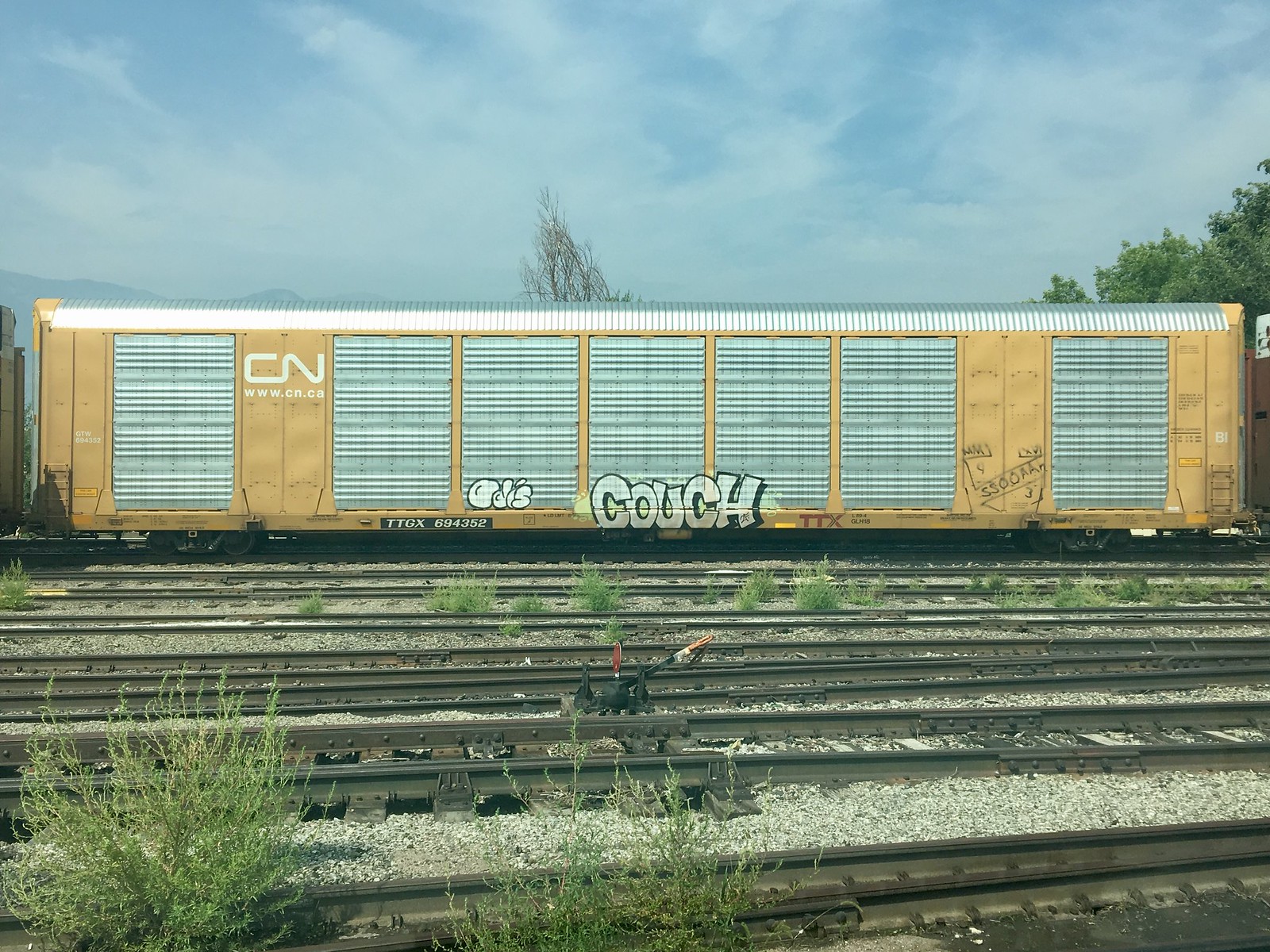This image features a bustling train yard with approximately six sets of train tracks stretching across the scene. The tracks in the foreground have patches of overgrown weeds and greenery, and occasional black debris is scattered among the tracks, lending a slightly neglected appearance. The central focus of the image is a yellow, brown, and silver train car positioned just above the midline, stretching from left to right. This train car, adorned with multiple metallic shutters, prominently displays the CN logo along with the website www.cn.ca on its side. Graffiti, notably the word "couch" in large white letters with black shadows, is sprayed near the bottom. Above the train car, the sky is a vibrant blue with scattered thin clouds, and the scene is framed by a mix of bare branches and green trees, hinting at an early spring day. In the distance, additional train cars and a faint outline of mountains can be observed, completing this detailed panorama of the train yard.